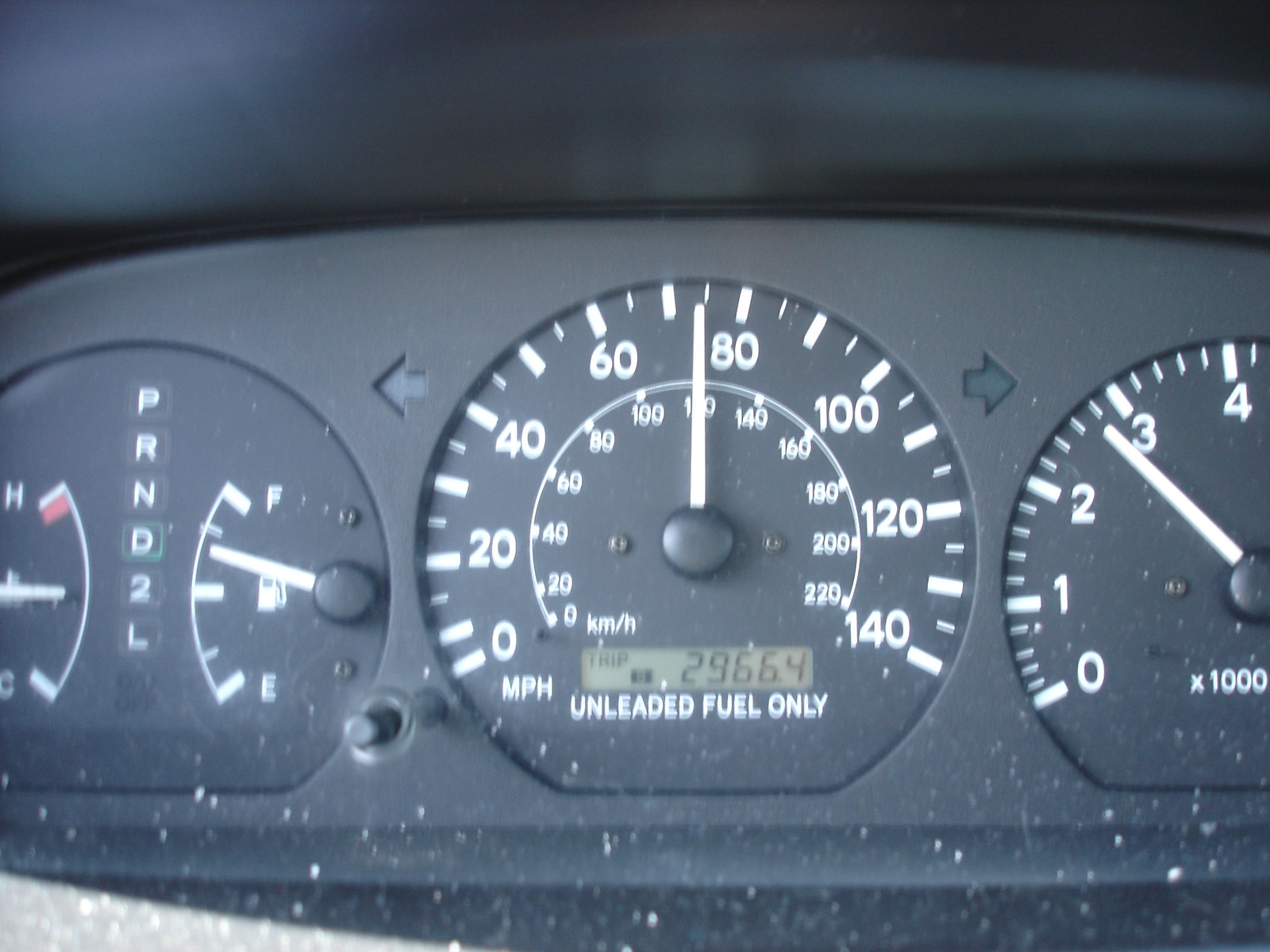The image presents a close-up view of a vintage vehicle's dashboard, prominently featuring three analog dials with white-font markings. On the far left, the first circular dial displays the engine temperature, with the needle positioned perfectly at mid-range, indicating an optimal temperature. This dial also shows the fuel gauge, with the needle resting at approximately three-quarters full, and an indicator for the gear selection, currently set to 'D' for Drive.

Centered in the trio is the speedometer, which measures speed in miles per hour and has a smaller, secondary scale for kilometers per hour. The speedometer's needle points to roughly 75 miles per hour. Just below the dial, a digital display indicates a vehicle mileage of 29,664 miles.

The rightmost dial, which is partially visible, monitors the engine's RPM. The needle is positioned just below the 3 mark, corresponding to around 3,000 RPM. The bottom of this dial carries a notation stating it measures RPM in multiples of 1,000. All numerical and textual information on the dashboard is displayed in a clean, white font, contributing to the classic, timeless aesthetic of the vehicle’s instrument panel.